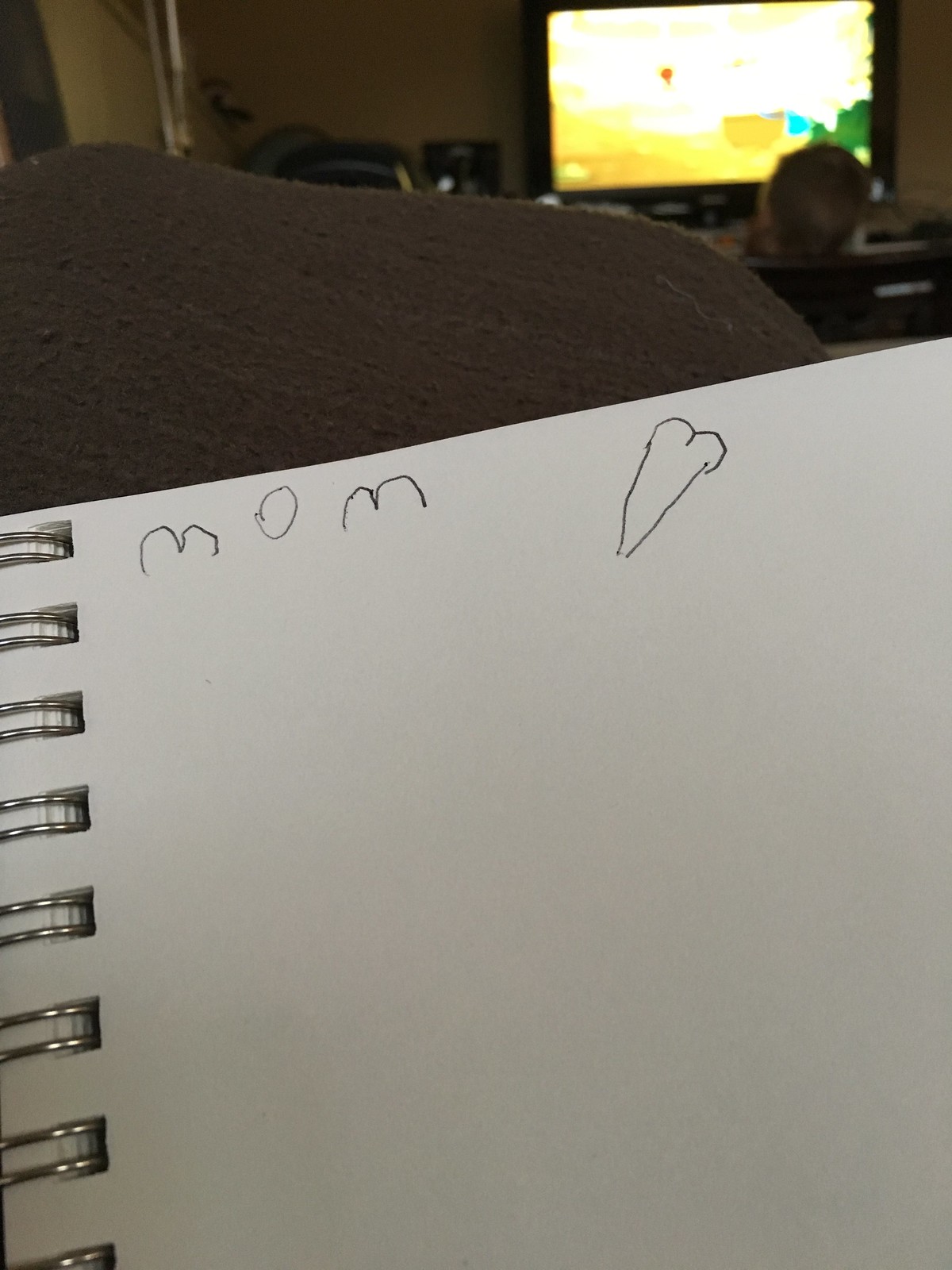The photograph captures a child’s heartfelt artwork in a spiral-bound notebook with a brown cover. The piece features a page of plain white paper bound with silver spirals on the left. At the top of the page, in slightly shaky handwriting indicative of developing motor skills, the word "MOM" is prominently displayed. Beside it is a drawing of a heart, though it vaguely resembles a carrot without a stem or leaf, showcasing two bumps at the top and a pointy bottom. The rest of the page appears blank from what is visible. The notebook seems to be resting on furniture adorned with a brown cushion above it. In the far background, a television screen, bathed in hues of yellow, orange, green, and blue, is faintly visible, though out of focus. Additionally, there are hints of other furniture pieces and possibly the back of someone's head in the background, reinforcing the intimate, homely setting of this tender moment.